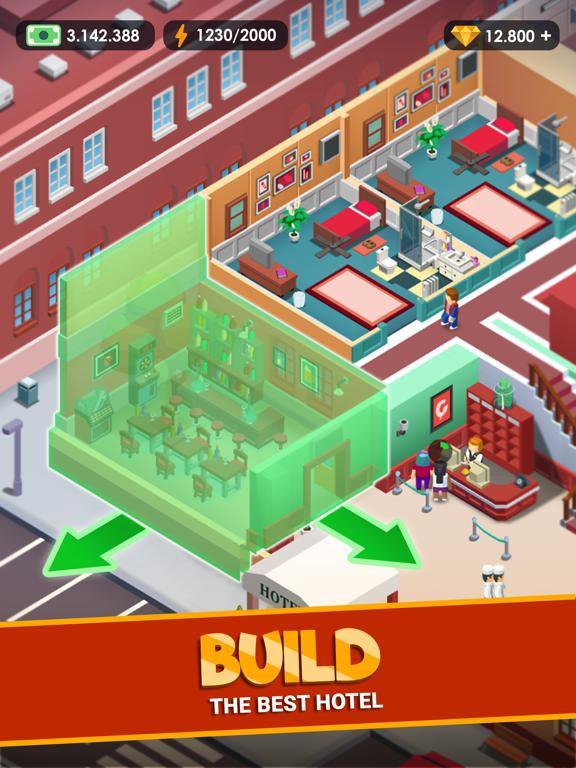This detailed and animated screenshot appears to be an advertisement for a cartoonish hotel-building video game. At the top of the screen, there are three distinct sections indicating different metrics: one with a money symbol, another with a lightning bolt, and the third on the right with a trophy and the number 12,800 with a plus sign. These likely represent various in-game resources such as energy levels or scores. 

In the center of the image, a large hotel is depicted with its roof removed, allowing a view into its interior. The hotel features multiple rooms with visible red beds and a staircase leading upward, creating a clear view of the layout. The lobby area, highlighted in green with arrows pointing in various directions, contains a reception desk behind which a lady is seated with two computers.

The bottom section of the image displays a thick orange banner with yellow and white text that says "Build the best hotel." This reinforces the game's objective and serves as an inviting call to action for potential players. Overall, the detailed and vibrant design elements, combined with the clear instructional text, effectively communicate the game's goal and interactive elements.